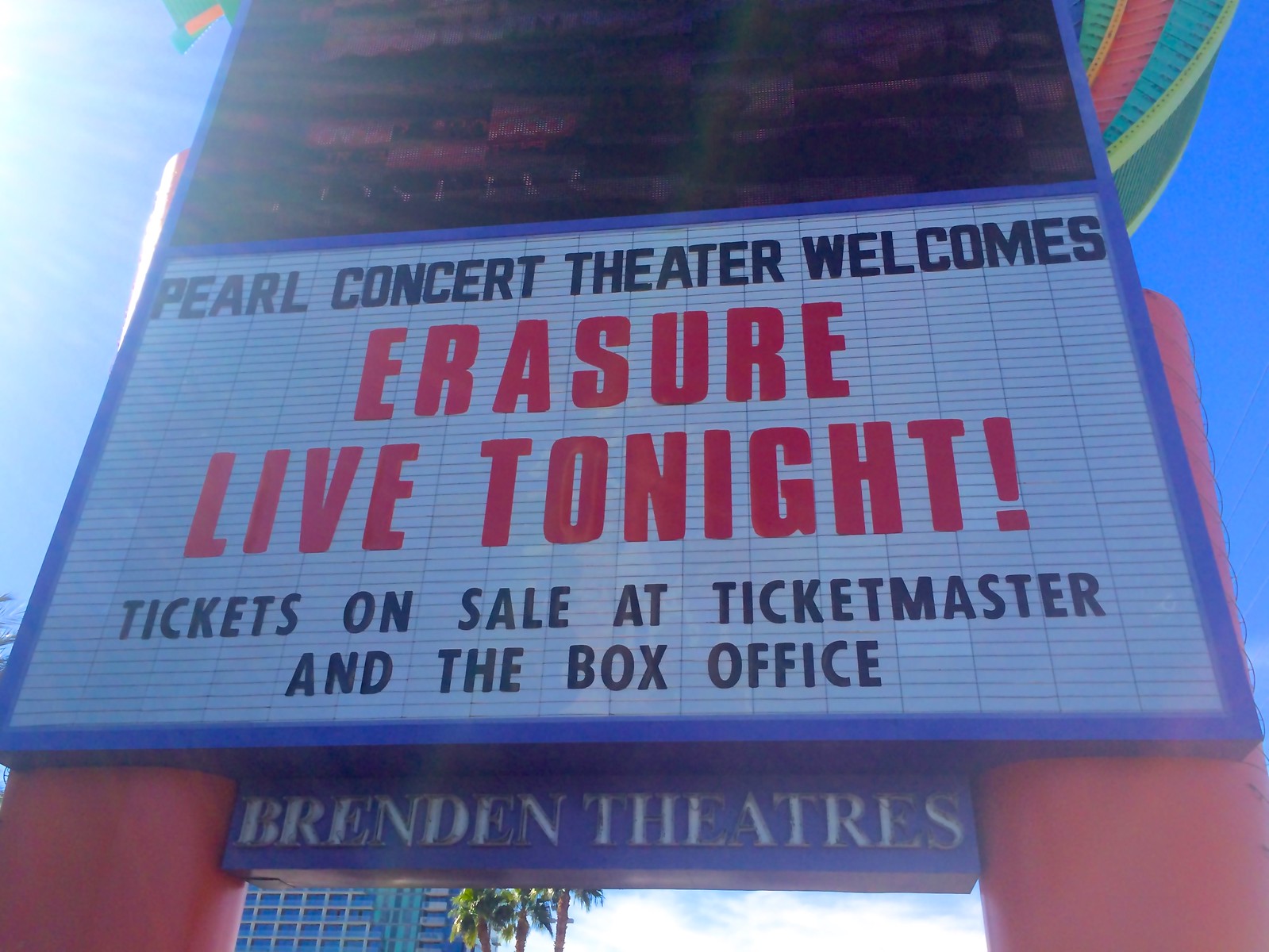The image showcases a towering marquee under a clear, sunny sky with visible sun rays on the left side. The marquee, framed in blue, has a white background with black letters at the top that read "Pearl Concert Theater Welcomes." Prominently displayed in the center are bold red letters announcing "Erasure Live Tonight." Beneath this, black text informs that "Tickets on Sale at Ticketmaster and the Box Office." The marquee is supported by two large red poles and has a rectangular section below it in blue lettering that reads "Brendan Theaters." Surrounding the sign are palm trees and part of a building, hinting at a lively and vibrant setting. The overall perspective of the image is from below, emphasizing the height and grandeur of the marquee.